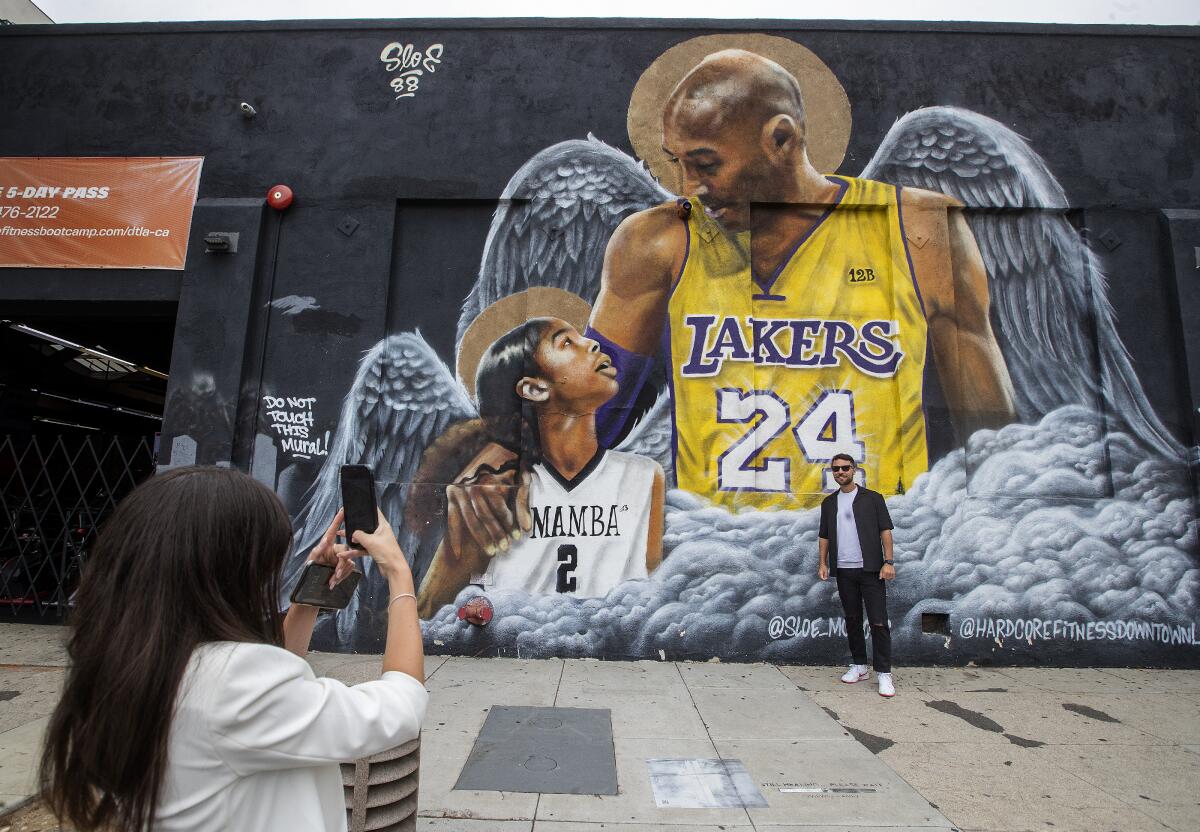This is a rectangular image of a mural painted on the side of a black building, commemorating Kobe Bryant and his daughter, Gianna. At the top, in white graffiti letters, it says "SLOE 88" and "do not touch this mural." The mural, against a backdrop of clouds, features Kobe Bryant, wearing a yellow Lakers jersey with the number 24, and large angel wings. He has his arm around Gianna, who is looking up at him, dressed in a white jersey that says "Mamba 2" and also has angel wings. Both figures have halos behind them. Standing in front of the mural is a man wearing sunglasses, a black short-sleeve shirt over a white shirt, dark pants, and white shoes. A woman with dark, long hair and a white jacket is taking his picture with a smartphone. The ground is concrete. The mural also has a small note at the bottom mentioning Hardcore Fitness.